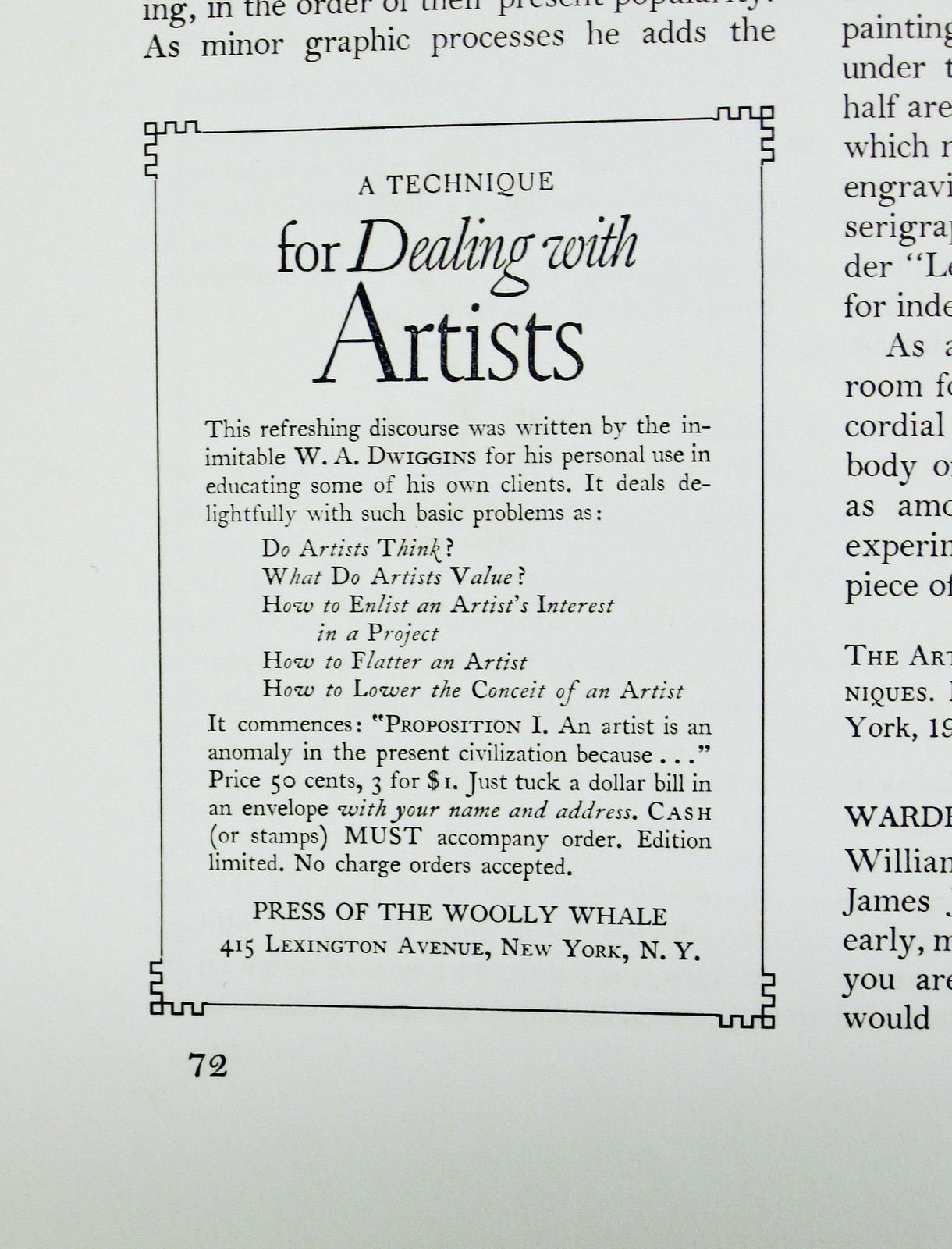This is a photograph of page 72 from a book or magazine. The layout is simple, featuring black text on a white background with a distinct border around it. The content starts with the title, "A Technique for Dealing with Artists," and continues with a refreshing discourse written by the inimitable W.A. Dwiggins for educating some of his clients. This piece covers various intriguing problems such as: "Do artists think?" "What do artists value?" "How to enlist an artist's interest in a project?" "How to flatter an artist?" and "How to lower the conceit of an artist?" It begins with Proposition 1: “An artist is an anomaly in the present civilization because...”

Additionally, there is commercial information: The price is listed as 50 cents or trade for 1 dollar. Instructions indicate to tuck a dollar bill in an envelope with your name and address, specifying that cash or stamps must accompany the order. Furthermore, the edition is limited with no charge orders accepted. The publication details include Press of the Woolly Whale, located at 415 Lexington Avenue, New York, NY.